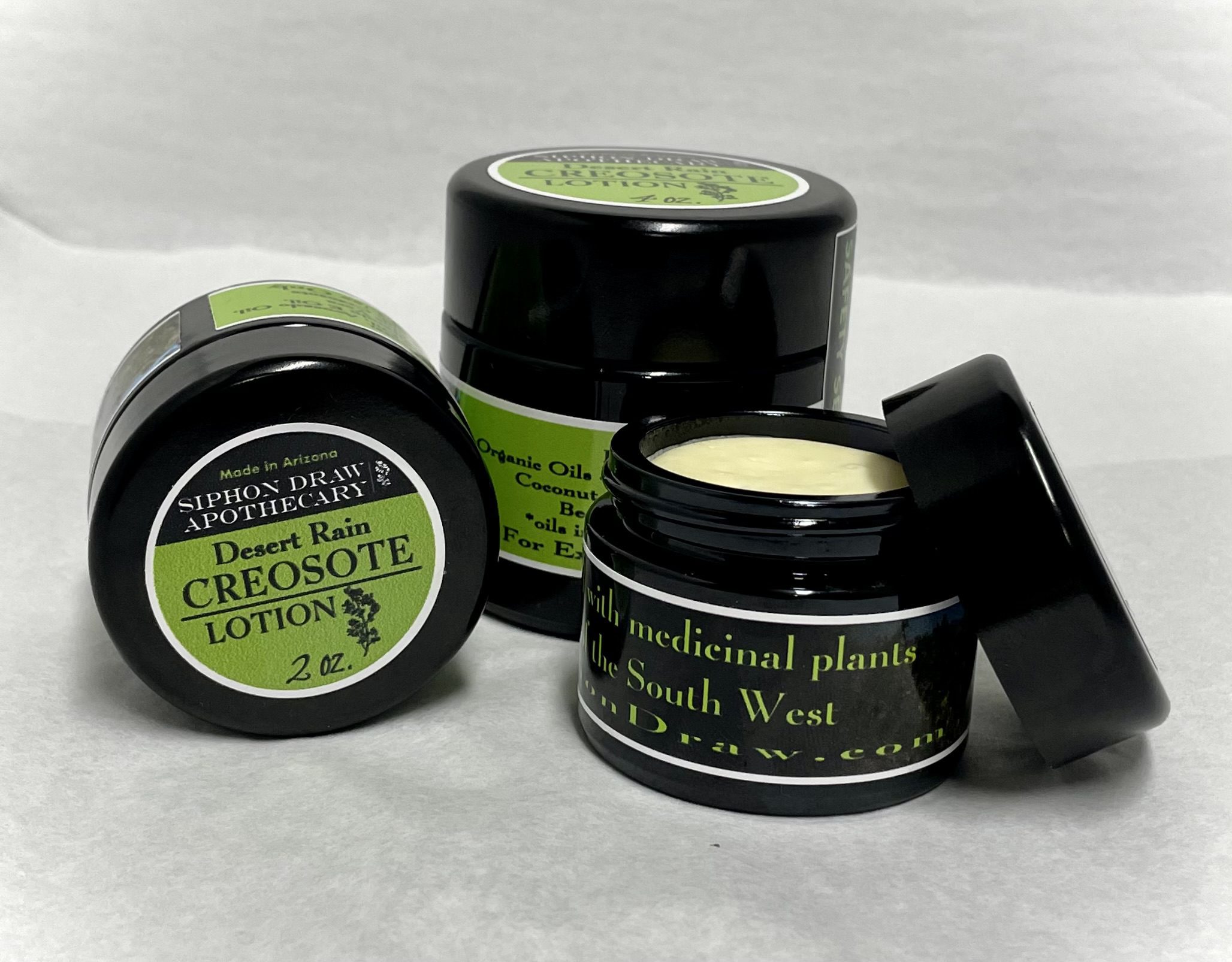This close-up photograph showcases three black cylindrical containers of lotion arranged on a gray fabric backdrop. The container on the left lies on its side, with the detailed label turned toward the viewer. The lid features a circular black top with an olive portion on the bottom, bordered by white. In olive and white text, it reads: "Made in Arizona," followed by "Siphon Draw Apothecary." The olive section includes black text: "Desert Rain Creosote Lotion," alongside "2-ounce" at the end. The centrally located, slightly taller container stands upright but has its text partially obscured; visible phrases include "organic oils" and "coconut." The rightmost container is also upright and open, revealing a white and beige lotion within. Its top is propped next to it. This container's label reads: "With Medicinal Plants," and includes "The Southwest" along with a partially visible website, likely ending in "draw.com." Each container shares similar design aspects, primarily consisting of green, black, and white hues on their labels. The overall presentation appears to be geared toward a product advertisement.